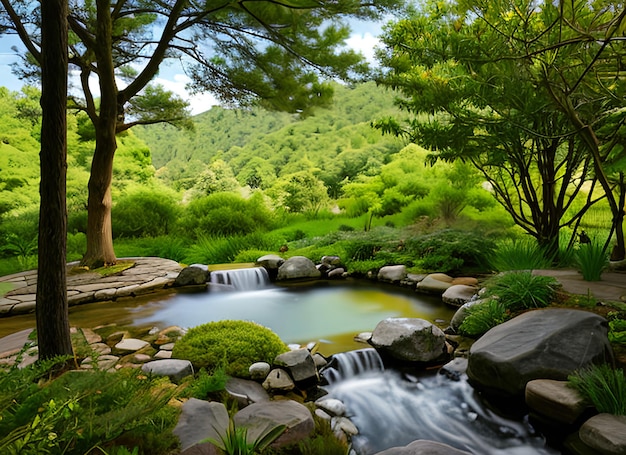The image appears to depict a digitally generated or heavily filtered outdoor scene that blends photographic realism with an artistic, cartoon-like quality. Dominating the scene is a small pond encircled by earthy brown boulders and rocks. The clear, blue stream cascades into this pond, creating white foam as it flows from both the upper and lower ends, giving the water a greenish tint as it pools amidst the stones. Surrounding the pond, lush green trees and foliage fill the landscape, with rolling hills and a blue sky adorned with white, puffy clouds in the background. To the left, a circular stone path wraps around the base of a tree, adding a man-made touch to the natural setting. The serene and tranquil atmosphere is accentuated by the absence of people and animals, making it a picturesque and inviting woodland or garden setting, perfect for peaceful contemplation.